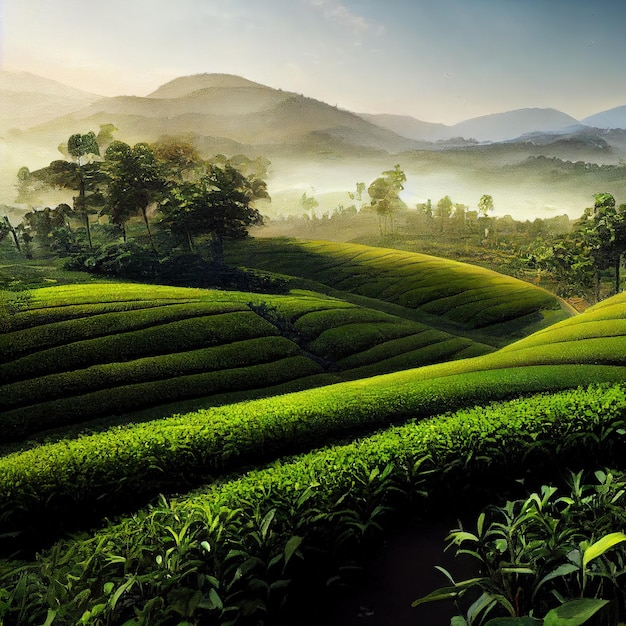The image depicts a serene rural landscape with a blend of lush green farm fields and rolling hills that evoke the charm of a realistic painting or digital art. The foreground showcases vibrant green fields that gently roll downwards and upwards, creating an undulating terrain of bumpy sections covered in short green plants. As the landscape progresses, it transitions into a patchwork of different agricultural plots, possibly growing various crops.

On the left, the fields transition into a dense patch of forest with tall, green trees and thick underbrush. Similarly, the right side has a cluster of more sparsely distributed trees, with a mix of yellowish-green foliage, indicating a different kind of vegetation. Beyond these verdant expanses, the background is dominated by towering mountains shrouded in clouds and fog, adding an ethereal quality to the scene.

The sky above is a tapestry of soft clouds, with rays of sunlight breaking through, giving the impression of a calm, early morning or late afternoon. This gentle illumination casts a warm glow across the entire landscape, heightening the painting-like quality of the scene. The overall effect is a harmonious blend of nature’s beauty, captured in artful strokes that emphasize the vastness and tranquility of the countryside.